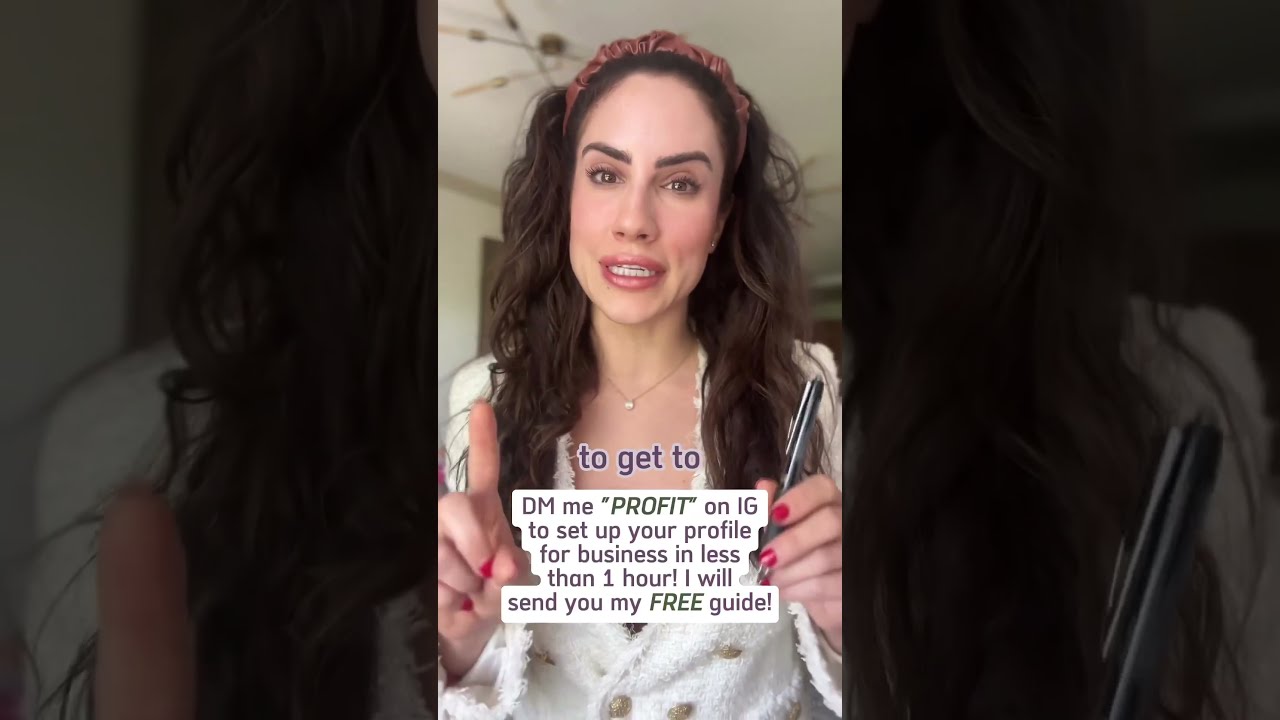The image is a screenshot of a woman with long, wavy brown hair extending beyond her shoulders, held back by a red headband. She appears to be in her 30s and is Caucasian. With thick brown eyebrows and red lips, she is visibly wearing red nail polish on her fingers. The woman, who is looking directly into the camera with a serious expression as if making an important point, has her hands raised to chest level, with her right hand holding a gray pen and her left hand's pointer finger raised. She is dressed in a white, fluffy-textured robe or coat that features tan buttons and a fringe, and underneath it, she wears a white vest. A delicate necklace with a jewel pendant adorns her neck. The background shows off-white walls and ceiling, suggesting an indoor setting, possibly her kitchen. Text overlay in the image reads: "To get to DM me quotes profit on IG to set up your profile for business in less than one hour I will send you a free guide," indicating it is an advertisement soliciting her business services.